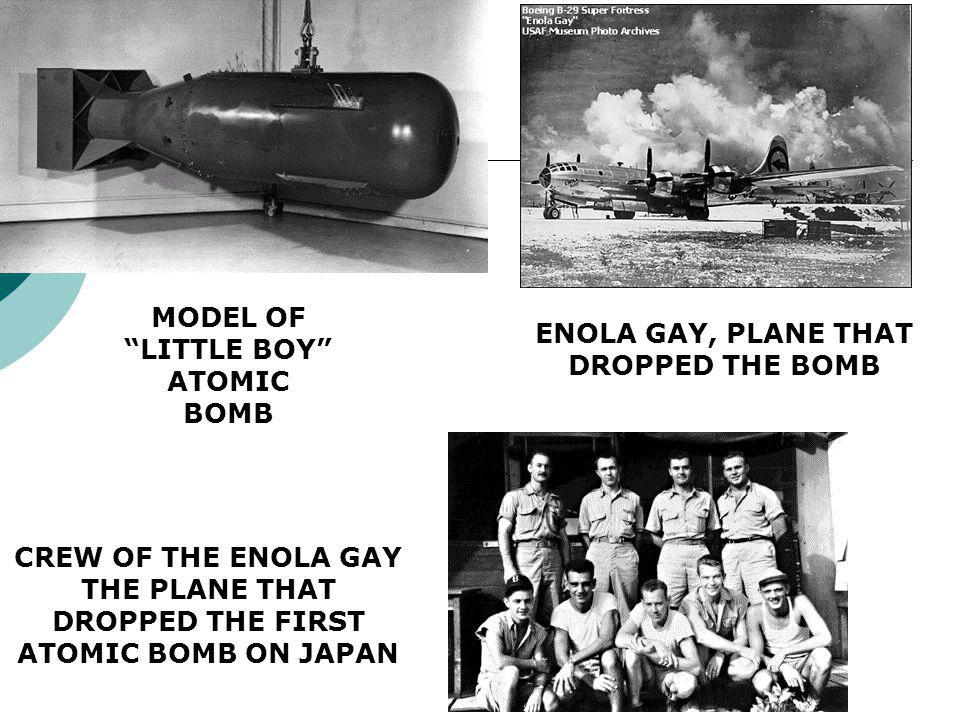The image is a detailed black and white collage related to the atomic bombing during World War II, comprising three distinct photographs and various descriptive texts. The top left section showcases an image labeled "Model of Little Boy Atomic Bomb," a representation of the bomb, which appears substantial in size. Adjacent to it on the right, there's a picture of a plane amidst clouds of smoke and water, identified as the "Enola Gay," the aircraft responsible for dropping the first atomic bomb on Japan. Beneath these, the collage features a photograph of nine men identified as the "Crew of the Enola Gay," posed and smiling for the camera. The accompanying text recounts their role as the crew of the plane that executed the bombing mission. The entire image, possibly intended for a magazine or news article, is set against a grayscale backdrop, contributing to a poignant portrayal of a significant wartime event.